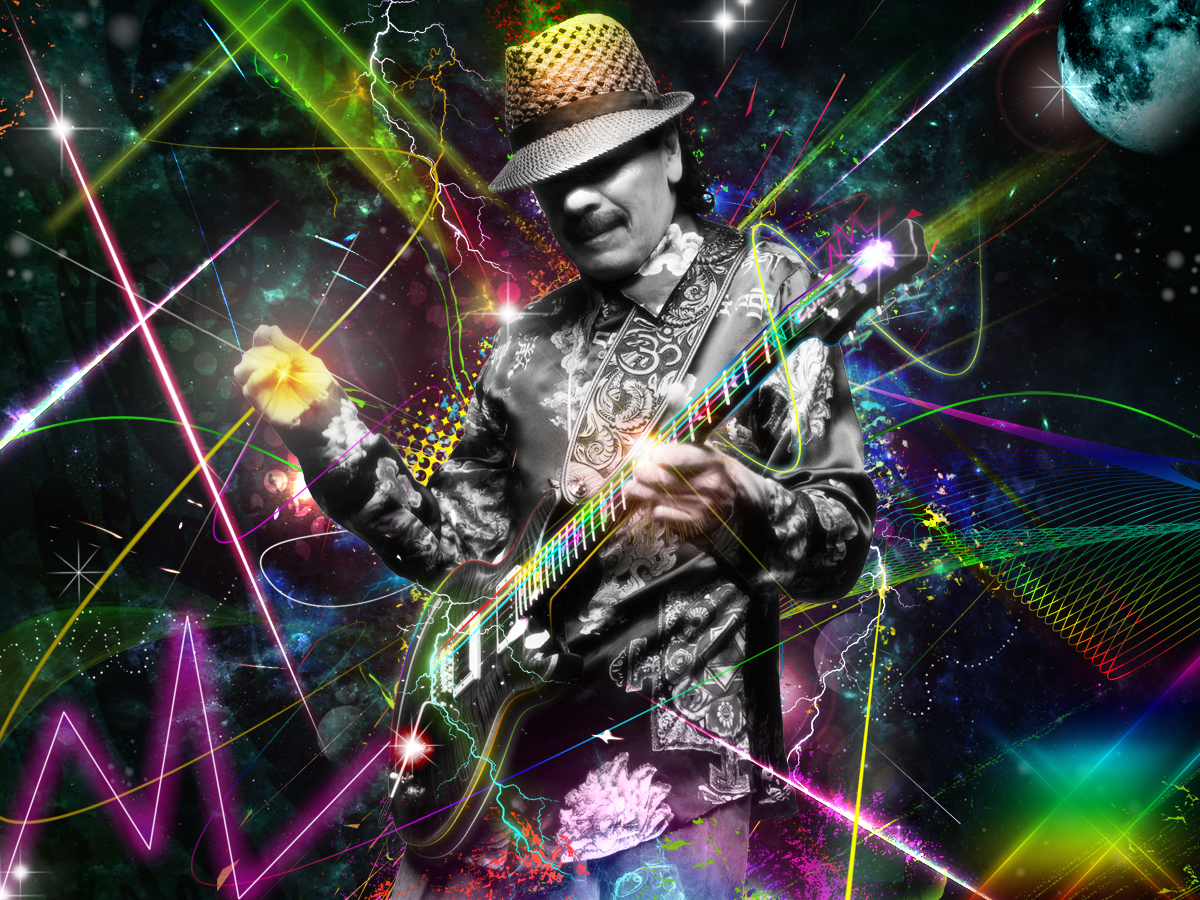The heavily edited photograph features a man immersed in a musical moment, holding a guitar. He is dressed in a striking black and white outfit adorned with intricate scroll-like patterns, and he sports a hat with a silver brim and a gold top, shading his eyes from view. His mustache adds to his distinctive appearance. The photograph captures him from his upper calves to the top of his head.

The background is an imaginative representation of space, dotted with small stars and featuring a heavily blue-filtered moon in the top right corner. Amidst the predominantly dark backdrop, vibrant lines and shapes electrify the scene. A pink zigzag brightens the bottom left, a radial rainbow line adds flair on the right, and yellow, purple, and red streaks are scattered throughout. Lightning bolts crackle towards the top, while a diagonal line cuts across from the top left.

The man's guitar strap is particularly eye-catching, with ornate designs, including the Hindu symbol for OM. The color saturation on the man himself is intensified, juxtaposed with the colorful chaos that surrounds him, making for a dynamic and surreal visual experience.